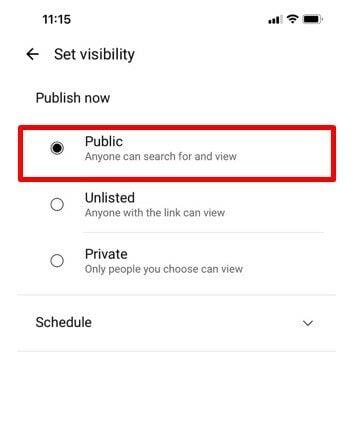The image capture appears to be a partially visible screenshot from a cell phone taken at 11:15, as indicated by the timestamp in the status bar. The phone shows three bars of network connectivity and a nearly full battery. The screenshot seems to be from an application where you can set the visibility of content before publishing it. 

At the top section, there's an option labeled "Set visibility," which is currently selected. Below this, there are three visibility options with corresponding radio buttons:

1. **Public**: Allows anyone to search for and view the content. This option is currently selected and highlighted with a red rectangle.
2. **Unlisted**: Allows only those with a direct link to view the content.
3. **Private**: Restricts viewing to a specific set of people chosen by the user.

Beneath the visibility options, there is a "Schedule" button with a dropdown arrow. Although the dropdown isn’t expanded in the image, this button likely allows the user to choose a specific date and time for publishing the content.

The overall design of the interface is simple and straightforward, focused on setting the visibility and scheduling the publication of the content.